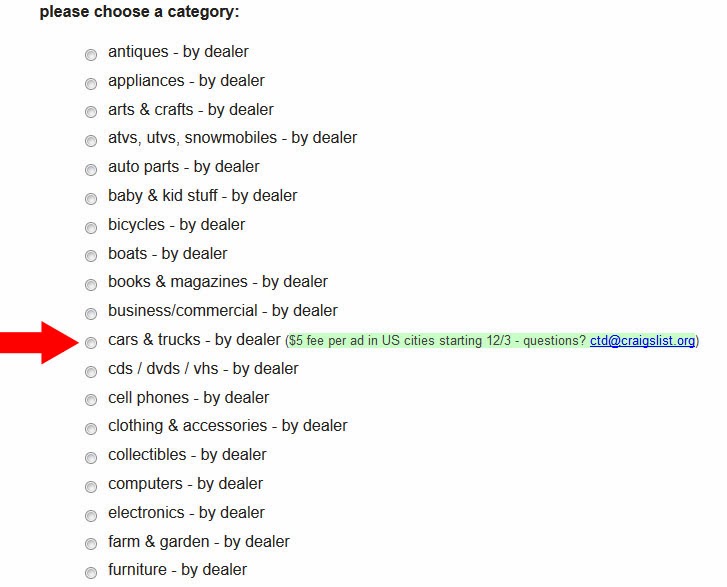This image is a screenshot of a categorized list, likely from an online advertisement platform such as Craigslist. The background is white with black font. A red arrow has been added to highlight a specific entry in the list. This arrow points towards the entry titled "Cars and Trucks – by Dealer." Next to this entry, there is a highlighted note stating: "$5 fee per ad in US cities starting at 12/3." Additionally, a blue, underlined link reading "CTD at Craigslist.org" follows this note, indicating an email link.

At the very top of the list, there is a header that reads, "Please choose a category:" followed by various item categories for dealers. The categories listed in order include: "Antiques – by Dealer," "Appliances – by Dealer," "Arts and Crafts – by Dealer," "ATVs, UTVs, Snowmobiles – by Dealer," "Auto Parts – by Dealer," "Baby and Kids Stuff – by Dealer," "Bicycles – by Dealer," "Boats – by Dealer," "Books and Magazines – by Dealer," "Businesses/Commercial – by Dealer," and the highlighted entry "Cars and Trucks – by Dealer." The list continues with "CDs, DVDs, VHS – by Dealer," "Cell Phones – by Dealer," "Clothing and Accessories – by Dealer," "Collectibles – by Dealer," "Computers – by Dealer," "Electronics – by Dealer," "Farm and Garden – by Dealer," and finally, "Furniture – by Dealer."

The screenshot captures these entries in a clear and organized manner, with the highlighted entry and corresponding notes standing out for easy reference.